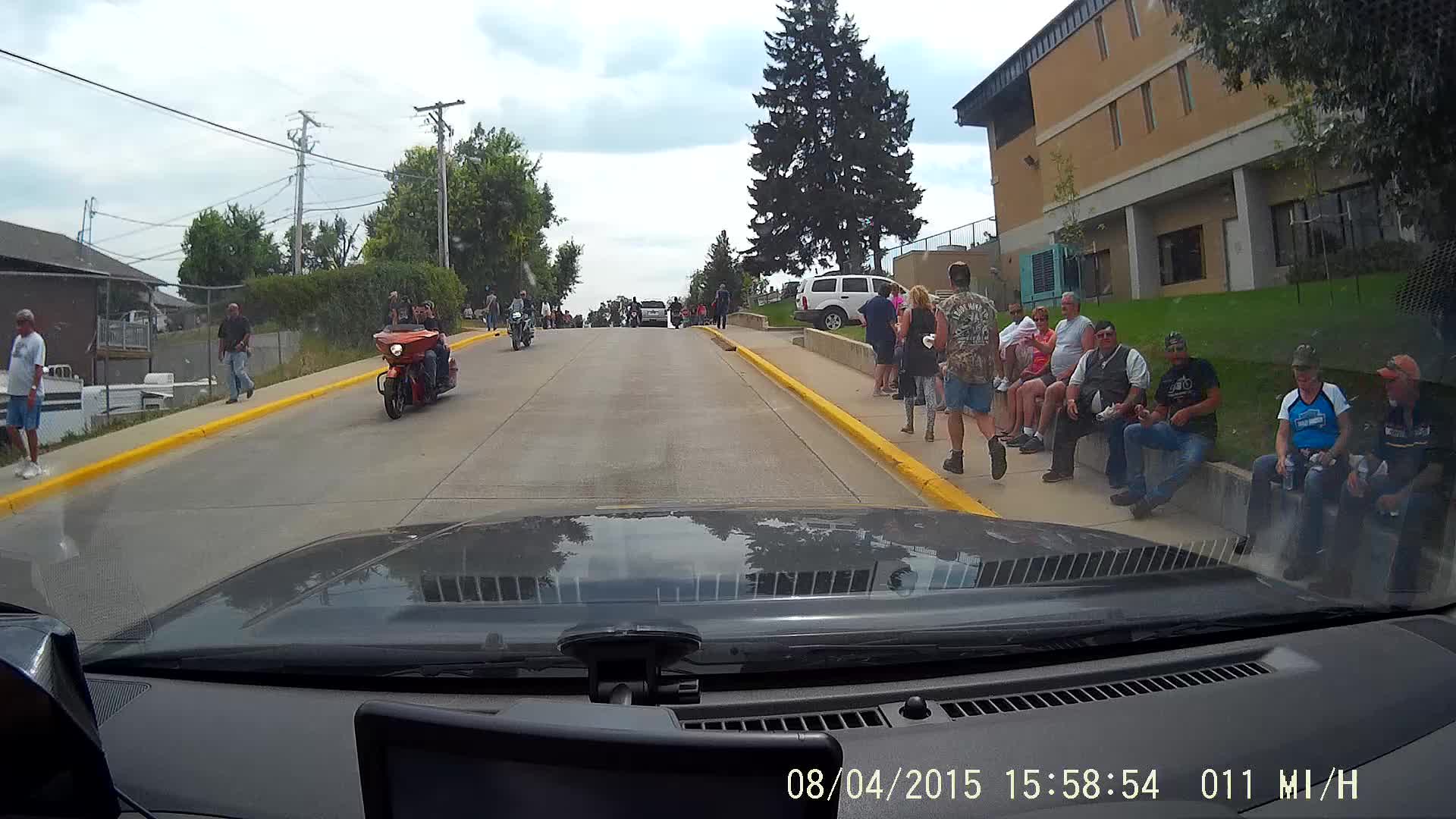A dash cam captures a snapshot from inside a vehicle, showing a gray hood and dashboard. In the bottom right corner, a timestamp reads "08-04-2015, 15:58:54," along with "011-M1-H." The scene outside features a light gray paved road flanked by yellow-painted curbs. An orange motorcycle approaches from the opposite direction, while pedestrians walk along the street. Approximately 10 to 15 people, dressed in a variety of colors including white, black, gray, and pink t-shirts, sit on a gray ledge with grass behind it. In the background, a brown brick building with gray accents frames the scene.